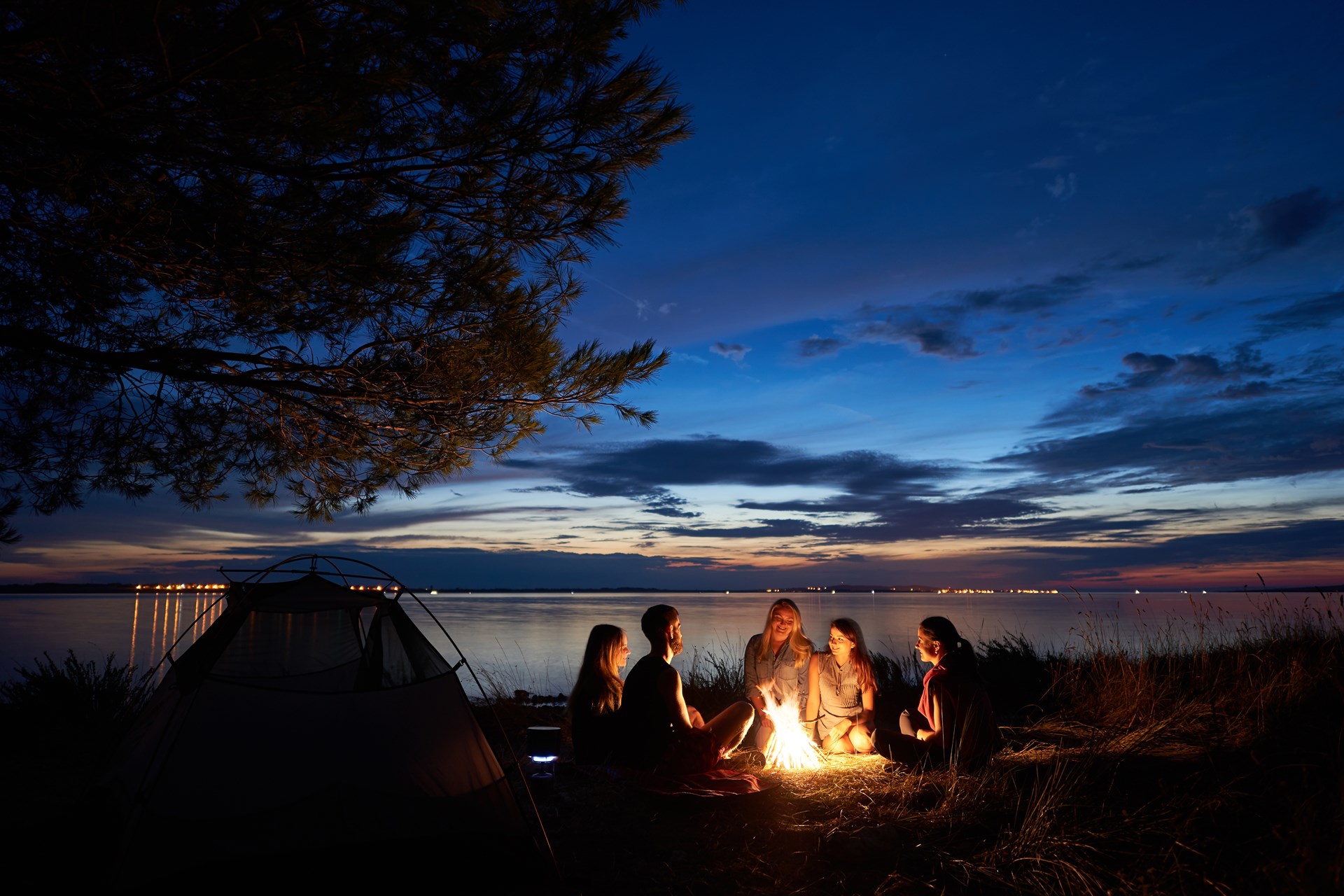This photograph captures a serene moment of five friends—four women and one man—gathered around a campfire near a large body of water, possibly a lake or river. The night sky is illuminated with a dusky palette of purplish-grey clouds, accented by hues of peach, pink, red, and yellow from the setting sun. The campfire, centrally featured with its large yellow flames rising from a teepee-stacked woodpile, casts a warm glow on the group. To their left, a dome-shaped tent is clearly visible, partially shaded by a brownish-green tree branch hanging in the upper left corner. The right side of the scene shows grass and reeds growing luxuriously. Across the water, yellow lights shimmer, adding to the calm ambiance. The quality of the photograph is quite good, with all elements in focus and well-lit, enhancing the beauty of this picturesque outdoor gathering.